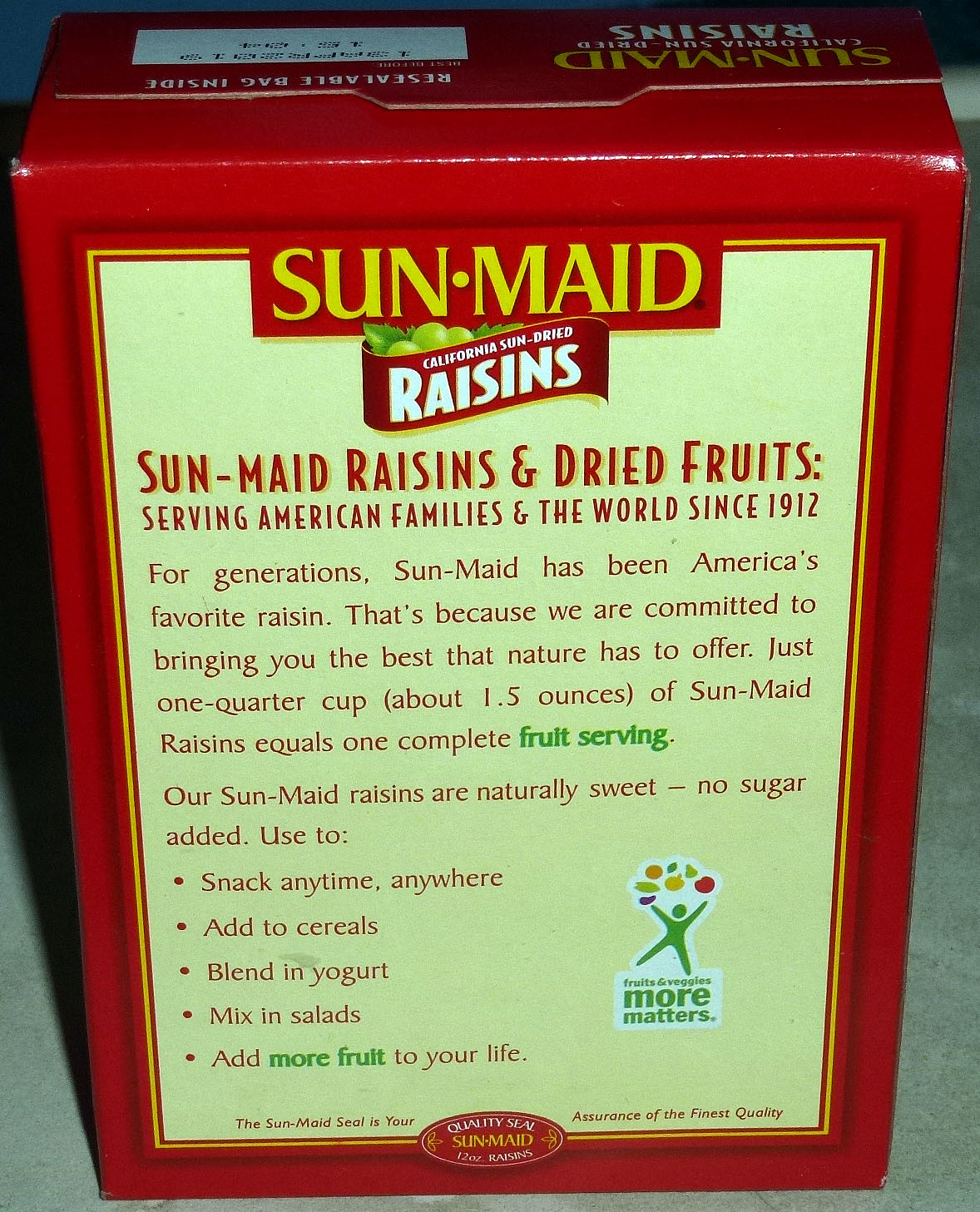This is a close-up color photograph of the back of a rectangular Sun-Maid raisins box, prominently filling nearly the entire frame. The box, standing on a smooth grey surface, is trimmed in red around the edges with an additional yellow border inside. At the very top, the Sun-Maid logo is displayed along with a banner that reads "California Sun-Dried Raisins" in white and "Resealable Bag Inside" in yellow.

Dominating the front is a large cream-colored label that states, "Sun-Maid Raisins and Dried Fruits: Serving American Families and the World since 1912." Below this, a detailed paragraph notes, "For generations, Sun-Maid has been America's favorite raisin. That's because we are committed to bringing you the best that nature has to offer. Just one quarter cup, about 1.5 ounces of Sun-Maid raisins equals one complete fruit serving." The label also emphasizes the natural sweetness of these raisins (with no added sugar), and suggests their versatility: "Use as a snack anytime, anywhere. Add to cereals, blend in yogurt, mix in salads, add more fruit to your life."

Towards the bottom right corner, there is a small logo depicting a green stick figure with arms outstretched, seemingly juggling colorful fruits. Underneath this image, there is some unreadable green text. Adjacent to this, at the bottom center of the box, lies another small oval logo with red writing, too tiny to discern. The box casts a subtle shadow to the left, enhancing the three-dimensional perspective of the image.